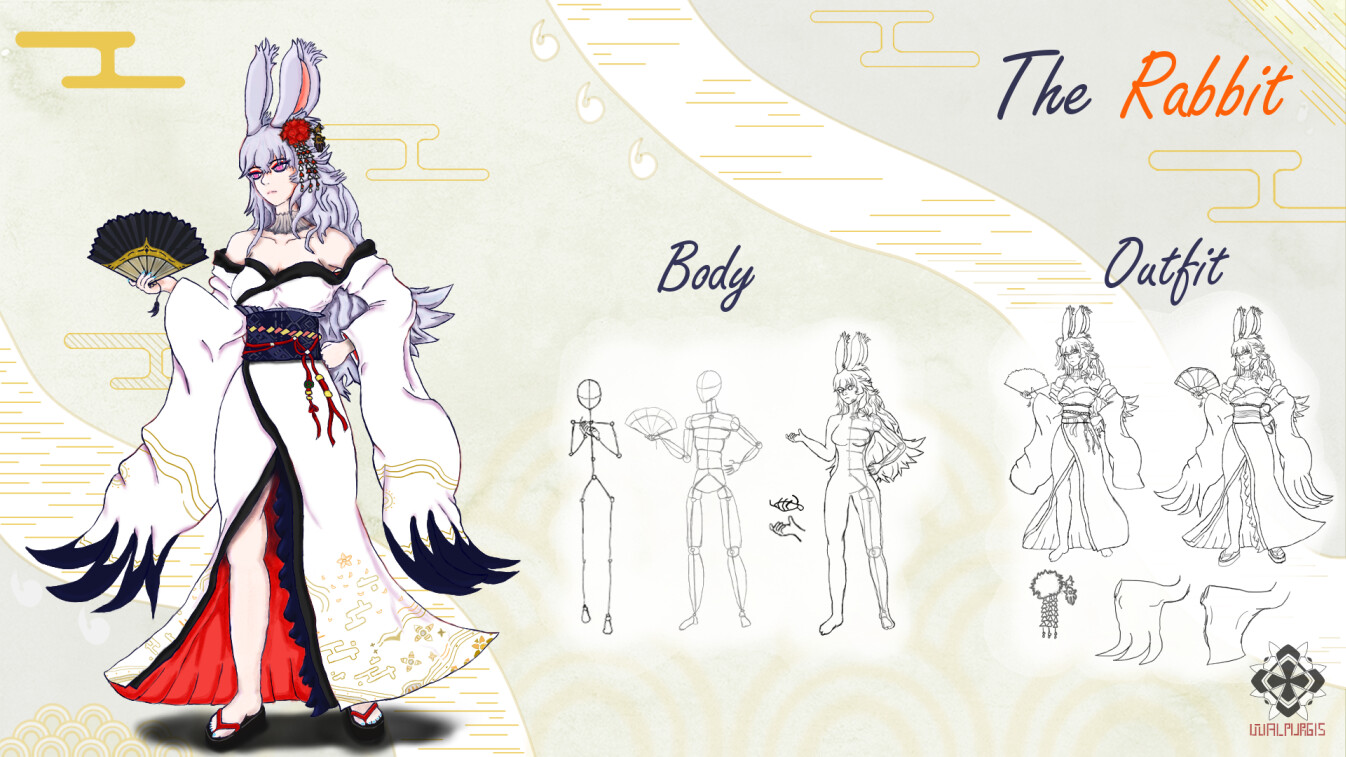The image is a highly detailed character design guide labeled "The Rabbit." Dominating the left side is the finished character, an elegant woman with long gray hair and matching rabbit ears, adorned with pink interiors. She wears a red flower in her hair and is dressed in an elaborate, eastern-styled, red and black dress. The dress, reminiscent of a Japanese kimono but tight-fitting and low-cut, features a high slit revealing her leg. She accessorizes with sandals and holds a fan trimmed in black.

Moving rightward across the image, we see a series of progressive sketches starting with simple outlines, labeled "body," showing how to form the character’s physique. Adjacent to these are more detailed sketches under the label "outfit," illustrating the development of the attire. Each sketch builds upon the last, ultimately leading to the fully realized, colored portrayal on the left. The background contains abstract graphic patterns, emphasizing the conceptual nature of the design process.